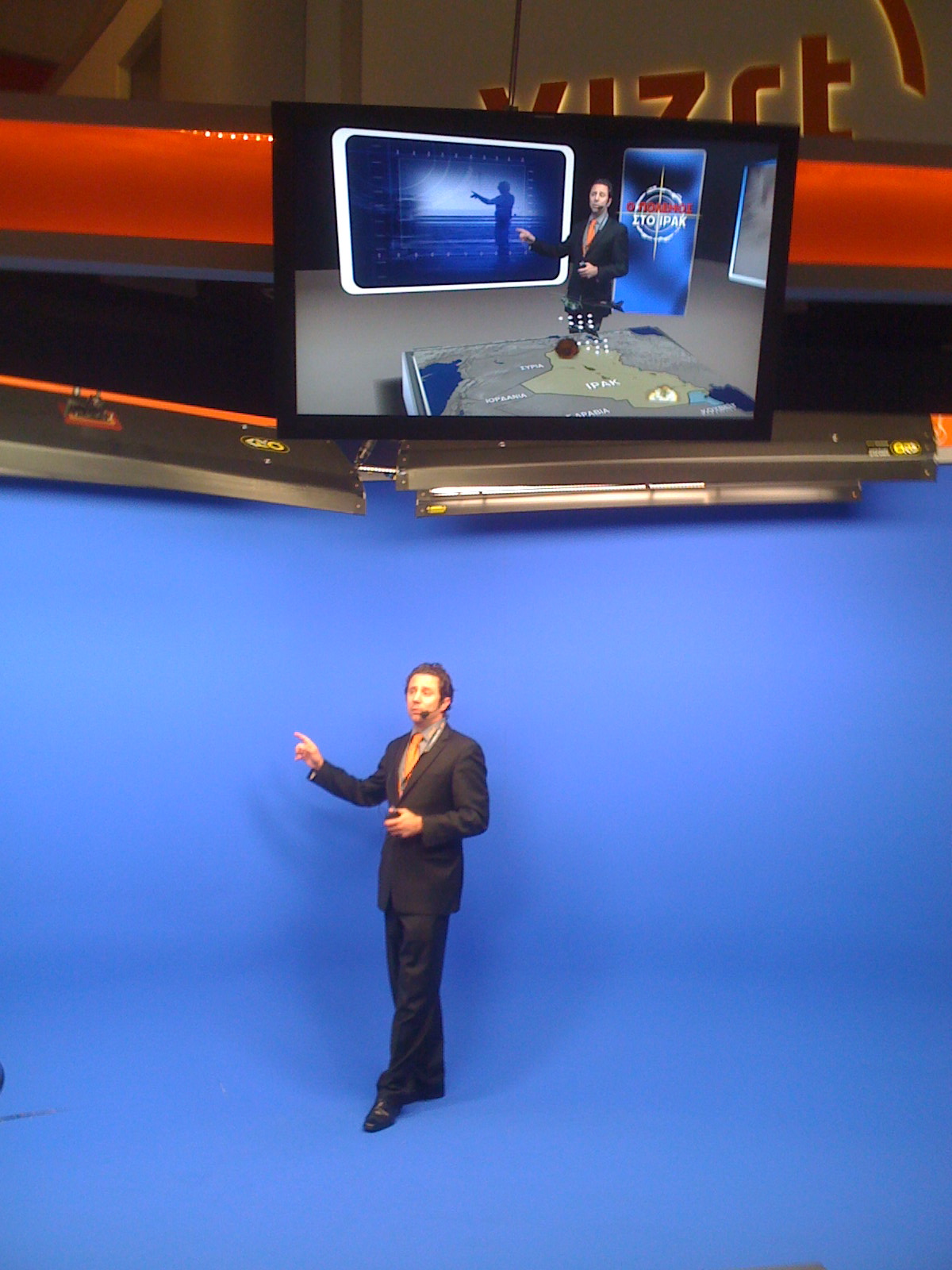The photograph captures a dynamic behind-the-scenes moment of a live newscast, with a portrait orientation. The bottom half of the image features a man in a black suit and orange tie, standing against a blue background. He is equipped with a headset microphone, suggestive of him being an on-air news presenter or possibly a meteorologist. The man has dark hair and is clearly engaged in delivering a report.

The top half of the photograph showcases a television screen showing the same man, but with additional visual elements superimposed. The screen image includes an orange and silver map behind him, hinting at a weather report, and there are indistinct letters and a logo indicative of a news channel, adding a professional touch. This composition illustrates the contrast between the raw setup of the blue screen backdrop and the polished, informative broadcast visible to viewers. The TV screen itself seems mounted on a wall, completing the busy newsroom environment. This detailed picture effectively merges the actual scene of the man standing against the blue screen with the enhanced visual of the on-air broadcast.